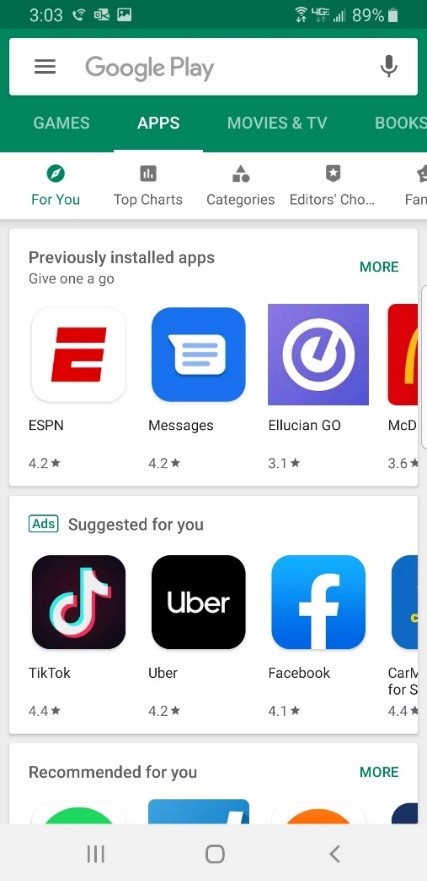This image is a mobile screenshot of an Android device, evident by the distinct navigation buttons at the bottom: a three-line icon (recent apps), a circle for the home button, and an arrow for the back button. The screenshot captures an outdated version of the Google Play Store, recognizable by its green header with a white search bar that reads “Google Play” and features a microphone icon for voice input. 

Below the search bar, there are various tabs for navigating different content categories: Games, Apps, Movies & TV, and Books, with the Apps tab currently selected. Within the Apps category, the user has navigated to the "For You" section. At the top of this section is a row displaying previously installed apps, including ESPN, Messages, Ellucian Go, and McDonald's. 

Further down, there is a section for suggested apps, including TikTok, Uber, and Facebook, which are marked as ads. Below the suggested apps, there is a "Recommended For You" section listing various app suggestions tailored to the user's preferences.